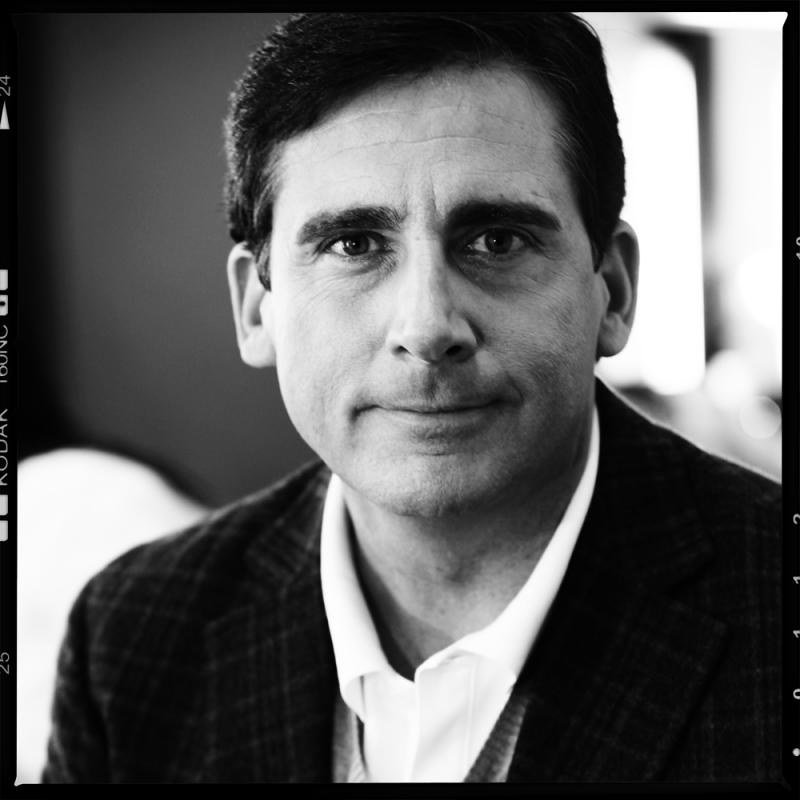The image is a black and white professional photograph featuring Steve Carell, the actor known for his role in "The Office" and various films. Steve Carell is centrally positioned and looking directly at the camera with a slightly confused expression tempered by a good-natured grin. He is Caucasian, likely in his 40s, with short, dark hair that tends to sweep to the right. He is dressed in a tweed suit coat over a white sweatshirt, adding a touch of casualness to his otherwise formal attire. The background is highly blurred, consisting of indistinct shades of white and gray, which further emphasizes Steve Carell as the sole focal point of the image. There are no visible texts, and the absence of clear background elements strengthens the impression that this is an indoor studio shot centered exclusively on Carell’s likeness.